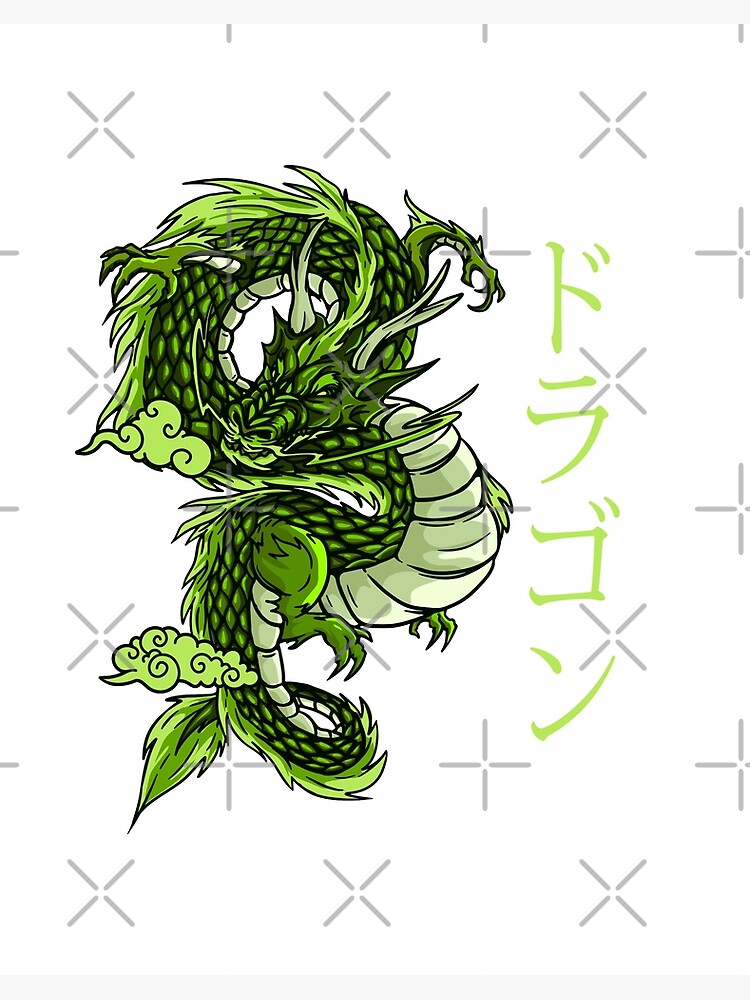This image features a detailed digital illustration of an eastern-style Chinese dragon, predominantly green in color. The dragon is depicted in a serpentine form, lacking wings but with a long, twisting body covered in green and black scales. Its underbelly is a pale green, transitioning to a tan shade in certain areas. The background of the image is white, adorned with light gray watermarks in the form of X's and pluses. The dragon's spine is lined with green fur that becomes a mix of lighter and medium green towards the tail. 

The dragon's face has an alligator-like shape, accentuated by long, swirling whiskers and greenish-gray antlers. Its expression is angry, and it is exhaling medium to bright green puffs of smoke, adding dynamism to the image. Four green kanji characters are positioned on the right side of the dragon, further emphasizing its cultural context. The overall effect is a vivid portrayal of the mythical creature, rooted deeply in ancient lore.